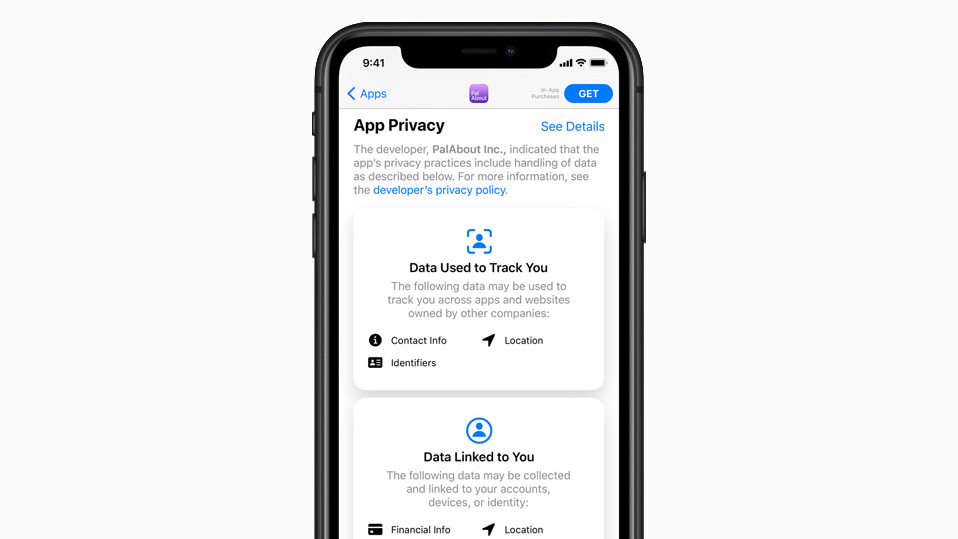Caption:

The image is a screenshot of a phone screen, surrounded by a medium gray border with three buttons on the left and one on the right, set against a light gray background. The phone's display shows a white background with the time "9:41" at the top, alongside internet icons and a battery icon. Below these icons on the left, there's a blue left-pointing caret followed by the word "Apps" in blue. Centered on the screen is a small purple square with text too small to read, flanked by a blue oval button labeled "Get" and the text "In-App Purchases" to the left of it.

Beneath this, the text "App Privacy" appears bolded in black, with "See Details" in blue to the right. Following this, it says "The developer, Palabout Inc. (P-A-L-A-B-O-U-T I-N-C.), indicates that the app’s privacy practices include the handling of data as described below. For more information, see the developer’s privacy policy," with "Privacy Policy" highlighted in blue, suggesting it is a clickable link.

Further down, there is an icon of a person within a blue square labeled "Data Used to Track You," followed by the statement "The following data may be used to track you across apps and websites owned by other companies." This section lists three categories: "Contact Info," "Location," and "Identifiers."

Below this, another icon of a person within a blue circle is labeled "Data Linked to You," with the note "The following data may be collected and linked to your accounts, devices, or identity." Visible in this section are categories for "Financial Info" and "Location," indicating that the list likely continues beyond what can be seen in the screenshot.